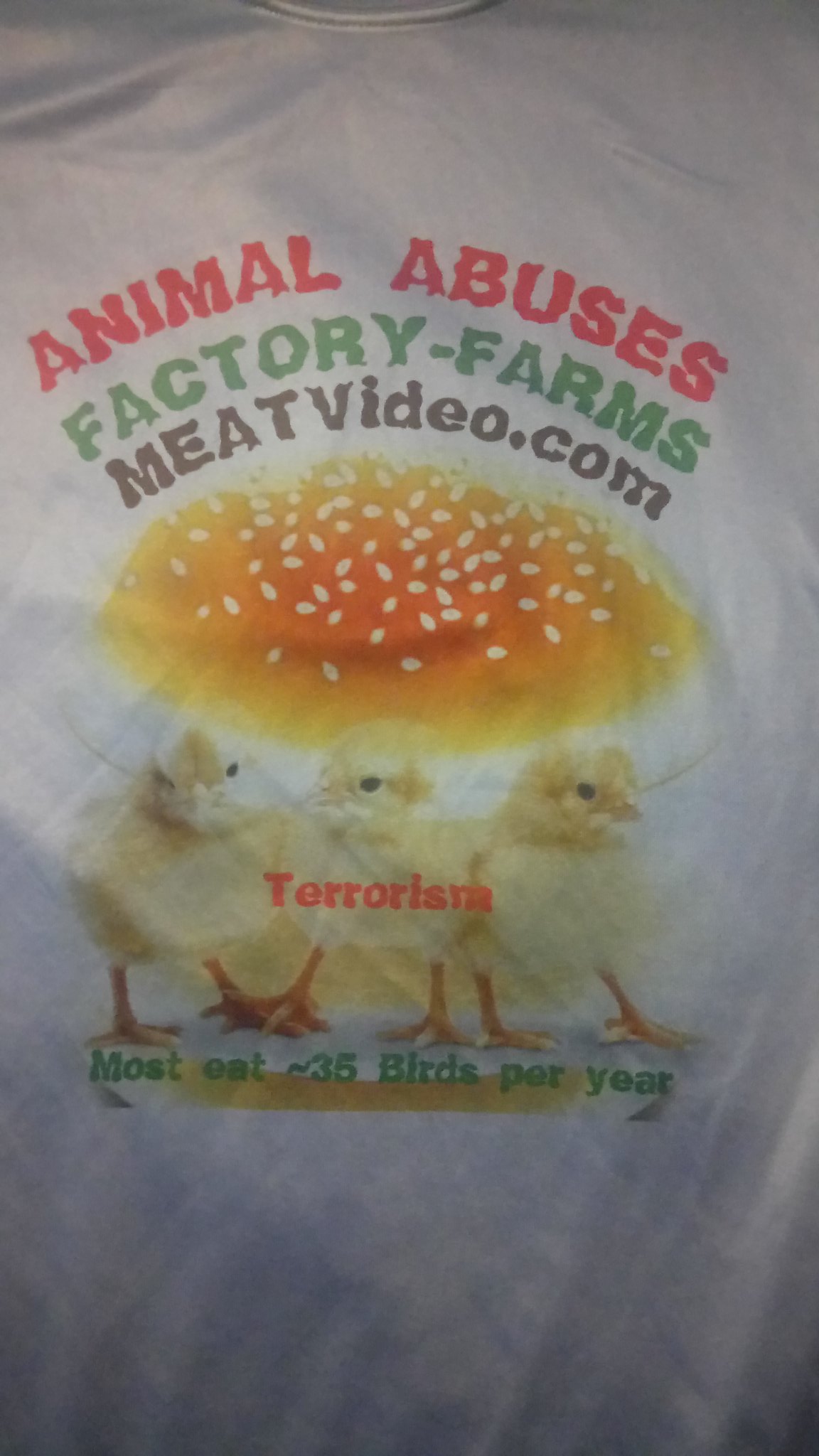This image depicts the front of a white t-shirt, featuring a slightly rippled surface with black shading at the bottom and visible neckline at the top center. The design is striking and impactful, beginning with bold red arced lettering that reads "Animal Abuses" at the top center. Just below, in green arced text, it states "Factory Farms," followed by "MeatVideo.com" in black, continuing the arced style. The central graphic includes the top bun of a sesame seed hamburger bun, placed above three small yellow chicks standing side by side, facing the right. Over their bodies, "Terrorism" is printed in prominent red letters. Below the chicks, in green text, it says, "Most Eat 35 Birds Per Year." The combination of the imagery and text creates a powerful message about animal abuse and factory farming.